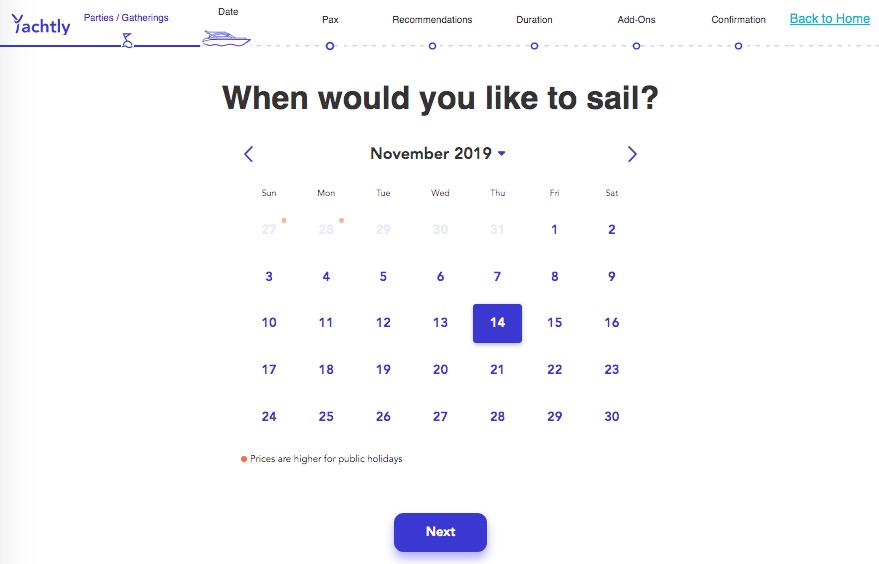This image is a left-to-right horizontal screenshot, likely captured from a website accessible via computer or smart device. The background predominantly appears white, transitioning to a grayish hue on the left-hand side, creating a clear contrast in this portion of the image.

In the upper-left corner, the text "Yachtley" is prominently displayed in purple. Directly beneath this, also in purple, are the words "party/gatherings" written on a small flag-like banner alongside a boat icon. Above this, in black, are several category headers: "Date," "Packs," "Recommendations," "Duration," "Add-ons," "Confirmation." There's a blue, underlined text labeled "back to home," likely functioning as a navigation link.

The boat icon appears to be traveling along a dashed line connecting various circles, which align under the respective black category headers mentioned above.

In the central white background, bold black text asks, "When would you like to sail?" Currently, the month displayed is "November 2019," with navigational arrows on either side for changing the month. Below this is a calendar, highlighting the 14th of November in purple. A key at the bottom of the calendar explains that red circles indicate higher prices due to public holidays. At the bottom right, a prominent purple button labeled "Next" invites further action.

The overall design is clean and functional, using color contrasts and navigational elements effectively to guide the user through the scheduling process.